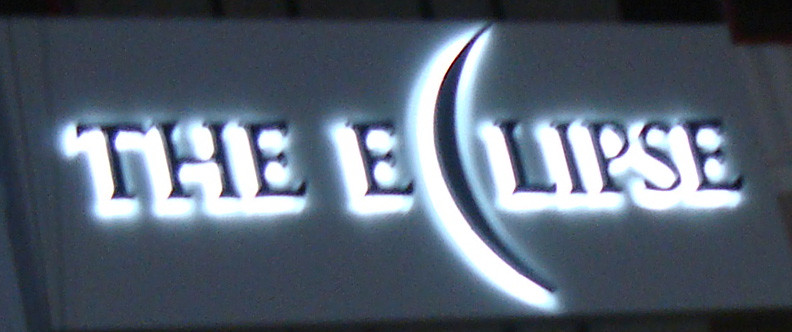The image is a stylized graphic or sign for a brand named "The Eclipse." The background features a charcoal gray color with a backlit appearance created by bright white fluorescent lights. The text, positioned centrally, consists of capital letters spelling "THE ECLIPSE." Unique to the design, the letter "C" in "ECLIPSE" is styled to resemble a crescent moon. The letters are rendered in dark blue or black with a white outline, providing a glowing effect that seems to cast a luminous shadow. The word "ECLIPSE" includes larger spacing and prominence, with the crescent "C" stretching from the top to the bottom of the text area. The image's orientation is notably horizontal, three times as wide as it is tall, and has the appearance of being out of focus. This horizontal format suggests the sign could be affixed to a building such as a hotel, captured at night under a dark sky.